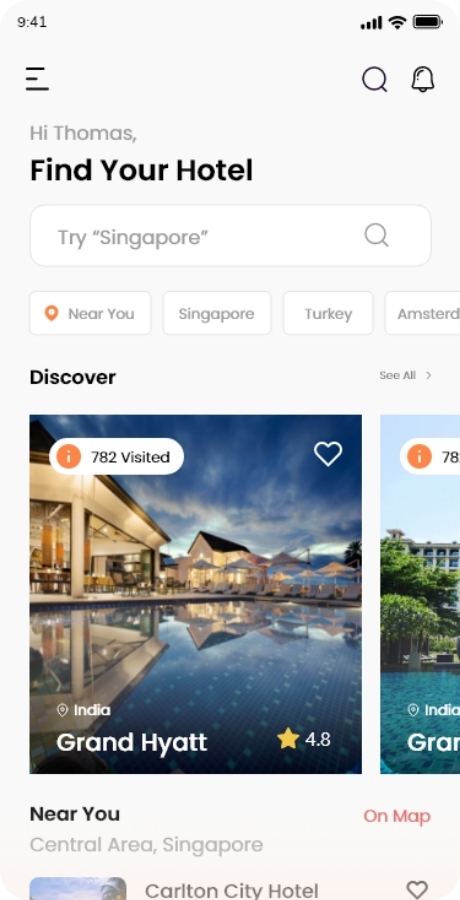The image depicts a cell phone screen showcasing a user interface for a hotel search application. 

At the top left of the screen, the time is displayed as 9:41. On the top right, there are icons indicating cellular connection, Wi-Fi connectivity, and a fully charged battery. Below this status bar, the screen is divided into several sections.

On the left of the next level is a tab menu. On the right side, there is a search bar followed by a notification bell icon. Beneath these elements, the user is greeted with the text "Hi Thomas" in black writing, with the prompt "Find Your Hotel" directly below it.

Following this greeting, another search bar is presented. Below the search bar, there is a horizontal white rectangle containing several categories organized from left to right: "Near You," "Singapore," "Turkey," and "Amsterdam."

Further down, the section titled "Discover" is displayed in black text with a "See All" option to its right. Below this, there is an image showcasing a hotel by or on a body of water, with the surrounding scene featuring a dark blue to gray-hued sky. In the top left corner of the image, an orange circle with "782 Visited" is displayed. The top right of the image showcases a heart icon. The hotel is identified as "India, Grand Hyatt" with a 4.8-star rating. 

Another hotel listing is partially visible to the right, displaying about 20% of its content. This fragment shows more water, trees, and a building in the background.

Directly beneath the main image, the text "Near You, Central Area Singapore on map" appears, followed by "Carleton City Hotel" at the bottom. The entire user interface has a light gray background.